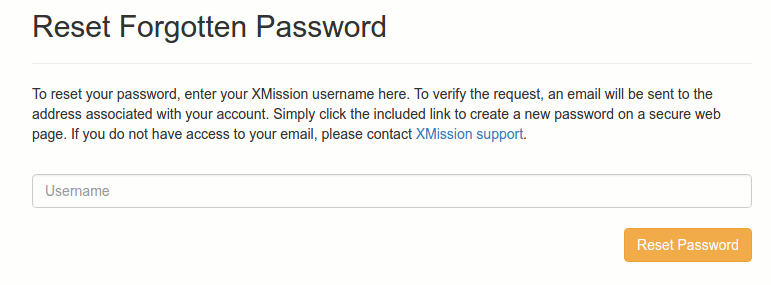The image displays a screenshot captured from a digital screen, focusing on a "Reset Forgotten Password" interface. Prominently, the interface features the phrase "RESET FORGOTTEN PASSWORD," with the R, F, and P capitalized for emphasis. 

The primary instruction states: "To reset your password, enter your X Mission username here." Following this, it explains that to verify the request, an email will be dispatched to the email address linked to your account. The email includes a link that you need to click to create a new password on a secure webpage. Should you lack access to your email, it advises contacting X Mission support, which is hyperlinked in blue text for immediate access.

Below these instructions, there is a white textbox outlined in gray, designated for entering the username. In the lower right-hand corner, there's a yellowish-orange button with the text "Reset Password" in white, inviting the user to proceed with the password reset process.